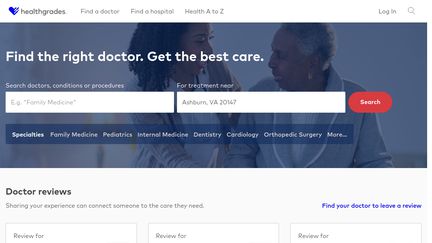Screenshot Description of Healthgrades Website

This screenshot captures the homepage of the Healthgrades website, showcasing its clean and user-friendly interface. The main header prominently displays the site's logo and tagline, "Find the Right Doctor, Get the Best Care." The top navigation bar features several tabs including "Find a Doctor," "Find a Hospital," and "Health A to Z," with additional icons for user login and a magnifying glass for search functionality.

Beneath the main banner, there is a search bar allowing users to input specific doctors, conditions, or procedures. Next to this is another text box labeled "For Treatment Center," where users can enter an address. A red "Search" button accompanies these fields.

A blue rectangular background section below the search area categorizes different medical specialties: "Specialists," "Family Medicine," "Pediatrics," "Internal Medicine," "Dentistry," "Cardiology," "Orthopedic Surgery," and an additional option labeled "More."

Directly underneath, there is a section dedicated to doctor reviews. The text reads, "Sharing your experience can connect someone to the care they need. Find your doctor to leave a review." Three empty text boxes labeled "Review for" give users the opportunity to submit their reviews.

The most prominent visual in the screenshot is a banner image at the top of the page. It features an African-American woman comforting an older African-American woman, symbolizing care and empathy.

Overall, the website aims to facilitate the search for medical professionals and encourage patient feedback to improve healthcare experiences.